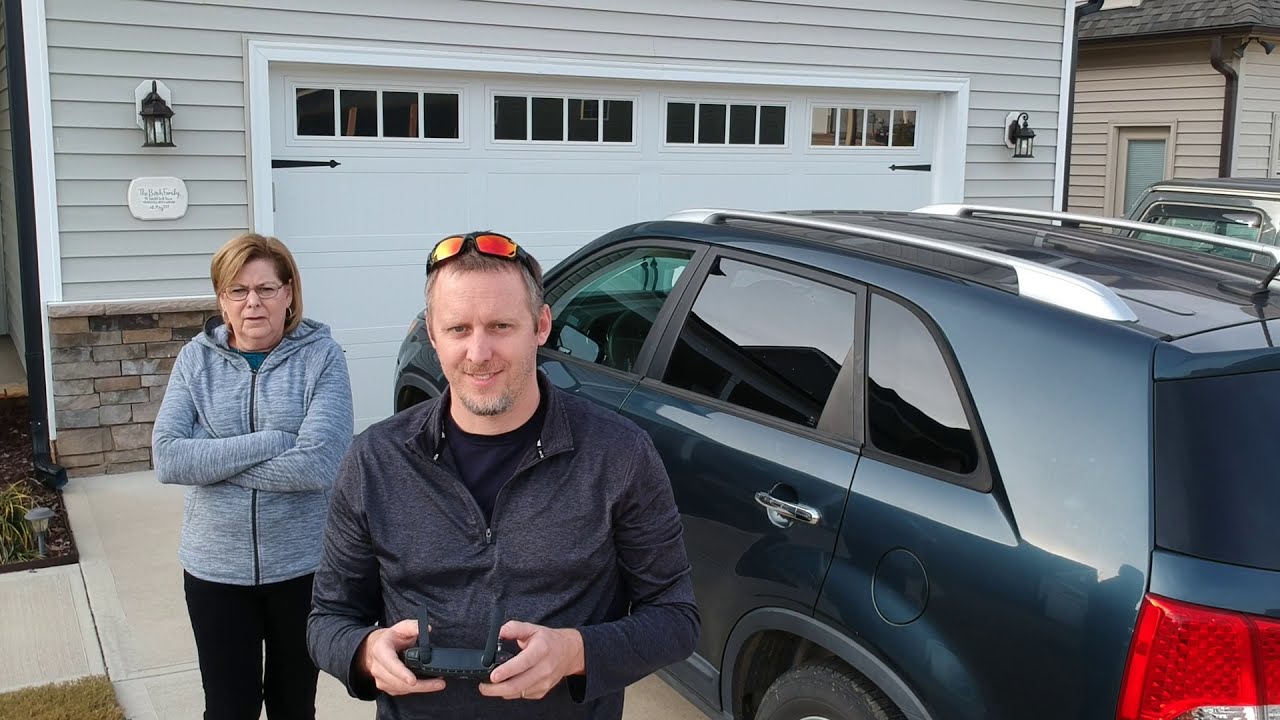In this detailed color photograph taken from a drone, a man and a woman are standing in a driveway in front of their home. The man, possibly aged 40-45, has short dark blonde hair and is wearing a very dark blue jacket over a navy blue shirt. He has orange sunglasses perched on his head and sports a scruffy beard. He is holding a remote control with two antennas, likely for a drone, and is looking up at the drone with a smile. To his left, slightly behind him, stands a woman who appears to be older, possibly around 65 years old. She has short dark blonde hair and is wearing eyeglasses, a light blue or gray zip-up hoodie, and black pants. Her arms are crossed, and she is standing on the sidewalk leading to their attached one and a half car garage. Parked in the driveway to the man's left is a dark blue or dark aqua SUV, resembling a Chevy Equinox, with a luggage carrier on top. The scene is set in front of their garage, with another home visible to the side. The photograph is a clear example of photographic representational realism, capturing a candid moment of what seems to be a shared experience of drone flying between the two individuals.